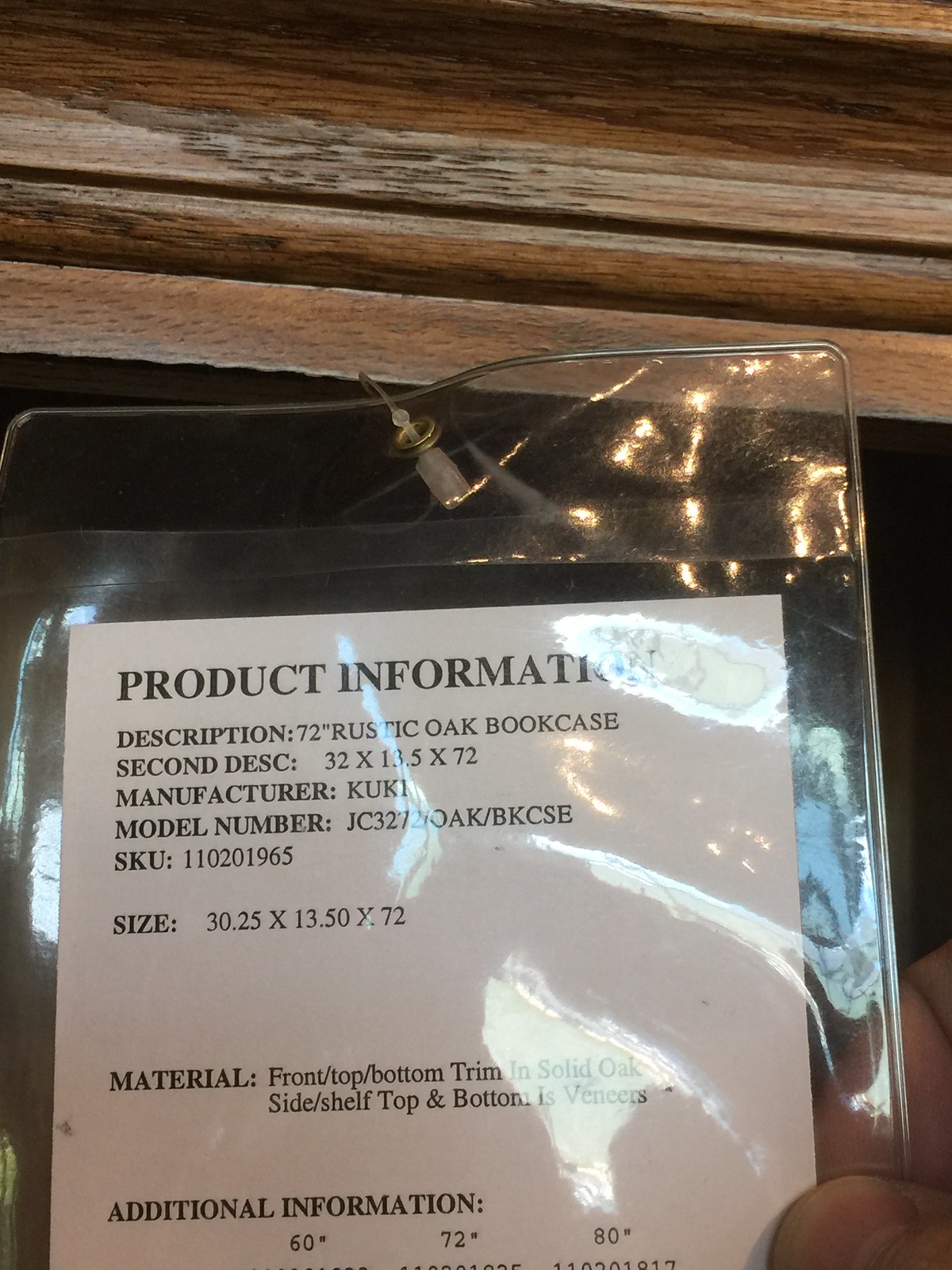This is a detailed photograph of a product information tag for a 72-inch rustic oak bookcase. The tag, a small sheet of white paper with black text, is encased in a clear plastic sleeve. It is being held in the lower right corner by someone's thumb and forefinger, barely visible in the image. The plastic sleeve, which has a reflective surface, is secured to the wooden bookcase by a plastic loop tie through a metal ring at the top.

The visible text on the paper provides comprehensive information about the bookcase, including its dimensions (30.25 inches by 13.5 inches by 72 inches) and materials used (solid oak for the front, top, bottom trim, and veneers for the side shelf, top, and bottom). Additionally, it lists the manufacturer, possibly spelled "KUKI" or "KUKK", and includes details like the model number, SKU number, and additional dimensions (60 inches, 72 inches, 80 inches). At the top of the tag, the heading reads "Product Information, Description: 72-inch Rustic Oak Bookcase." The wooden bookcase can also be seen in the background, particularly along the upper edge of the photograph.